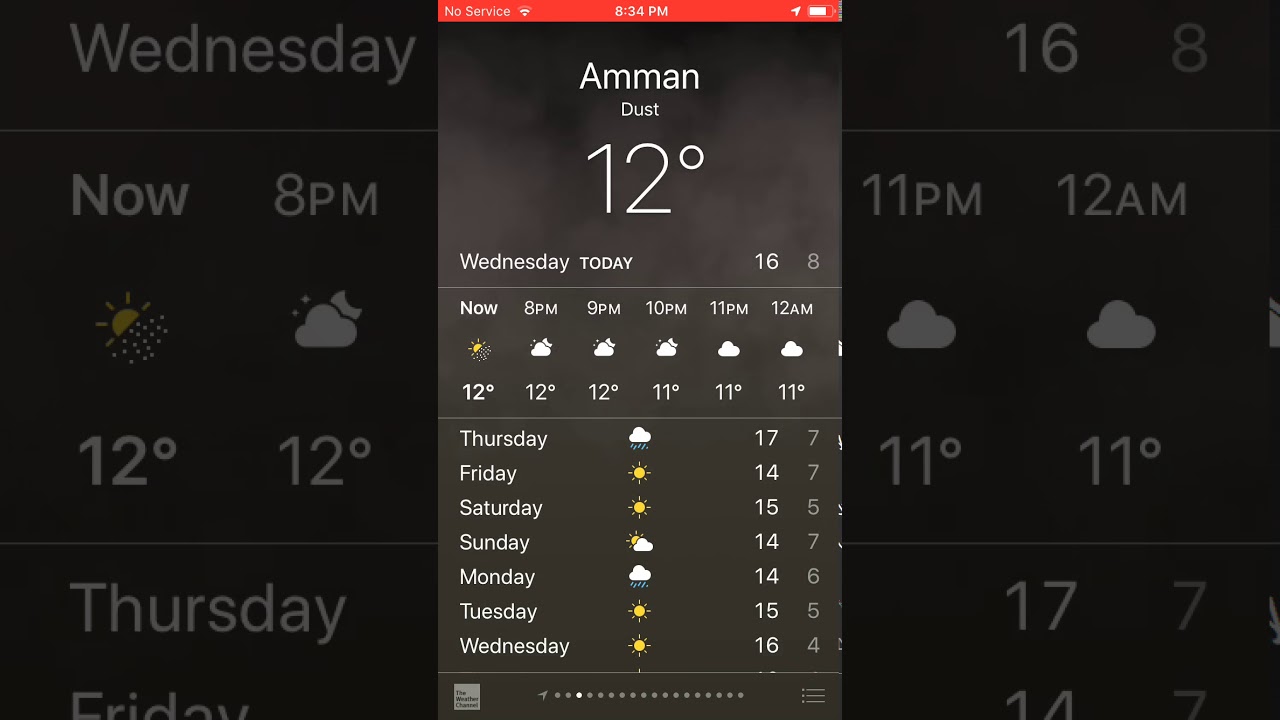In the center of this image, there is a zoomed-in view of a cell phone screen displaying a detailed six-day weather forecast. The top of the screen shows standard phone indicators: "No Service" in the top left corner, a Wi-Fi icon, "8:34 p.m." in the center, and a battery percentage bar in the top right corner. 

Directly below these indicators, it states "Wednesday Today," followed by a detailed hourly forecast from 7 p.m. to 12 a.m. Temperatures for the first three hours are all 12 degrees, dropping to 11 degrees for the final three hours.

The weekly forecast is presented beneath this, spanning from Thursday to Wednesday. Each day is represented by corresponding weather icons:
- Thursday: Cloudy with rain
- Friday: Sunny
- Saturday: Sunny
- Sunday: Cloudy
- Monday: Rain
- Tuesday: Sunny
- Wednesday: Sunny

The highest temperatures for each day, listed to the immediate right of these icons, are 17, 14, 15, 14, 14, 15, and 16 degrees respectively. Below each high, the lows are indicated: 7, 7, 5, 7, 6, 5, and 4 degrees.

Surrounding this central display, the left and right sides of the image replicate the phone screen’s hourly and daily forecasts but in a much more zoomed-in view, set against a black background.